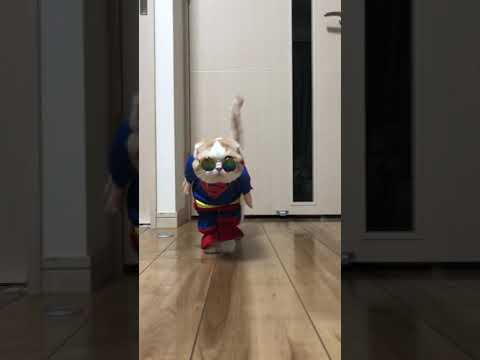In this vertical, borderline-free photograph, a white cat with short ears and a gray tail struts confidently towards the camera, seemingly embodying a little human figure due to its comical attire. The cat, standing on a beige wooden floor in an indoor setting with white walls and a white door in the background, sports a pair of sunglasses and an adorably mismatched costume. The outfit, designed to mimic a superhero, features a blue shirt with a red chest patch, and red and blue pants that appear only on the front legs. This amusing portrayal makes it look as if the cat has tiny arms and is walking upright like a little human. The various hues in the image—shades of white, tan, brown, red, blue, and yellow—add to the vibrant and playful nature of the scene, evoking a sense of satire often associated with viral content on platforms like TikTok.